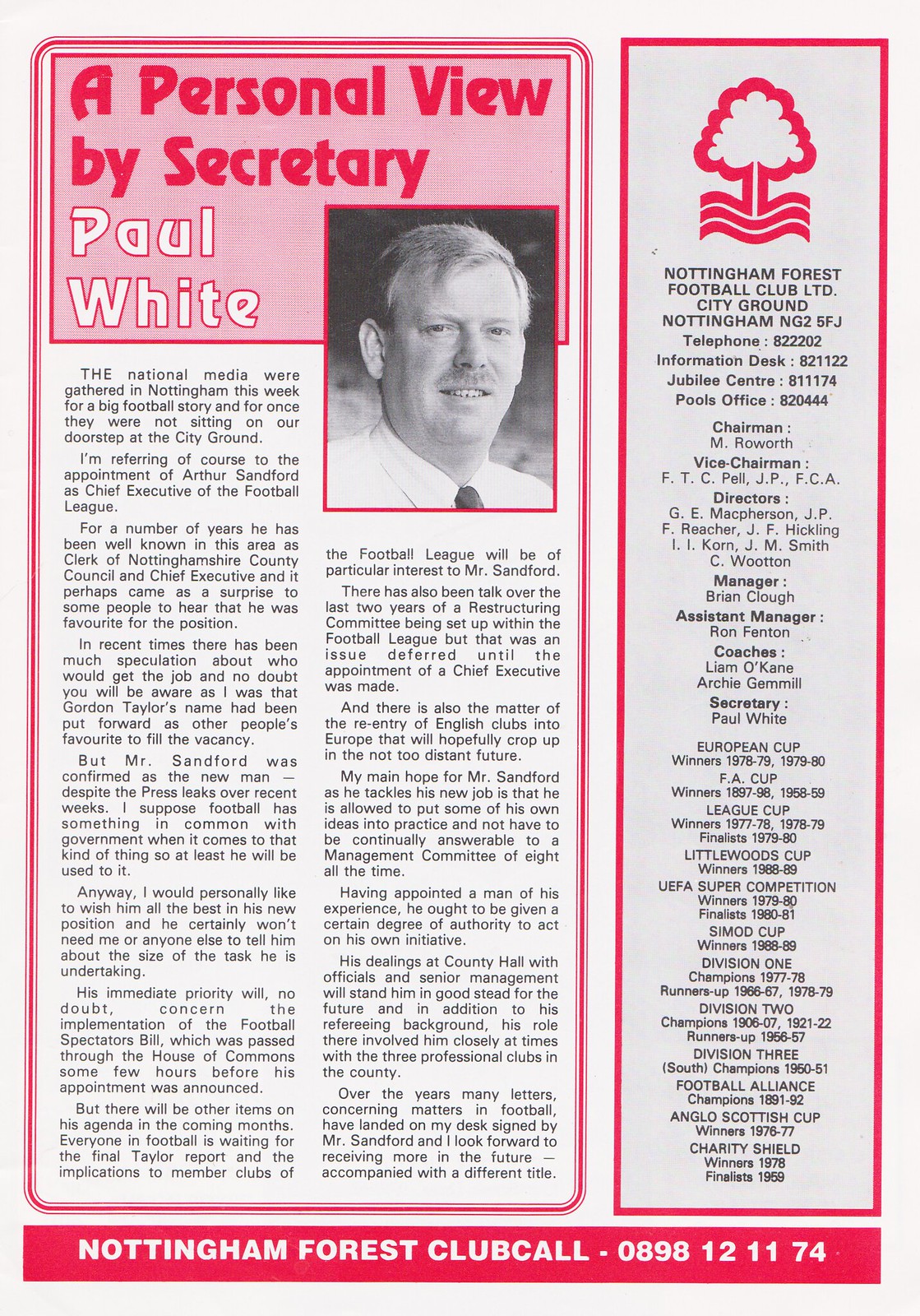The image depicts a page from a program or magazine, featuring two pink-bordered rectangles. On the left side, the rectangle contains a detailed article titled "A Personal View by Secretary Paul White," with "Paul White" written in white letters and the rest of the title in pink. Below the title, there is a lengthy article with black text thoroughly discussing the recent appointment of Arthur Sanford as Chief Executive of the Football League. Adjacent to the title, on the right side, is a black-and-white photograph of a person who is either Paul White or Arthur Sanford.

The right-side rectangle, positioned at the top, includes a drawing of a tree with waves underneath it. Below this drawing, there is text reading, "Nottingham Forest Football Club Limited, City Ground, Nottingham NG2 5FG, Telephone 822202," followed by additional contact information and a list of names. 

At the bottom of the image, there is a small horizontal pink strip, upon which white text reads, "Nottingham Forest Club Call 0898-121174." The overall design and setting suggest that this is a page from a sporting event program or magazine, with colors including tan, purple, white, grey, and black.